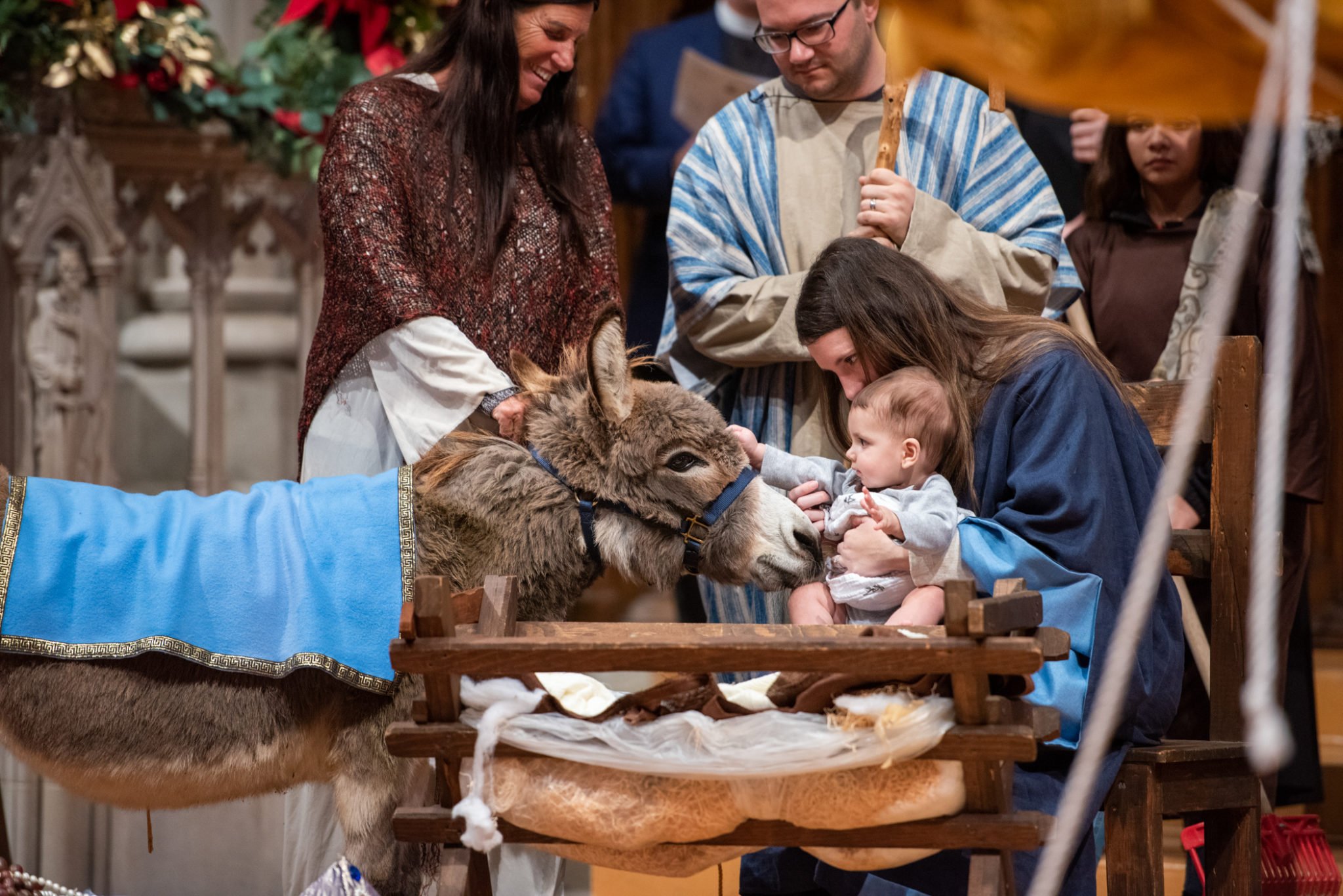In this detailed scene of a nativity, a serene outdoor setting features key figures gathered around a wooden manger. At the center, a woman draped in a blue robe cradles a baby dressed in diapers and a light blue shirt, while another woman, partially obscured and with long hair, tenderly encourages the baby to reach out and pet a donkey. The donkey, adorned with a blue blanket trimmed in silver, nudges gently at the baby's belly, exhibiting a calm demeanor. Completing the tableau, a man and a woman stand in the background. The woman, in a burgundy or brown dress, holds the donkey by the collar with a smile, while the man beside her, clad in a blue and white striped robe and holding a shepherd's crook, gazes down at the touching interaction with a soft expression. Blankets strewn in and around the wooden manger add to the rustic, heartwarming setting.